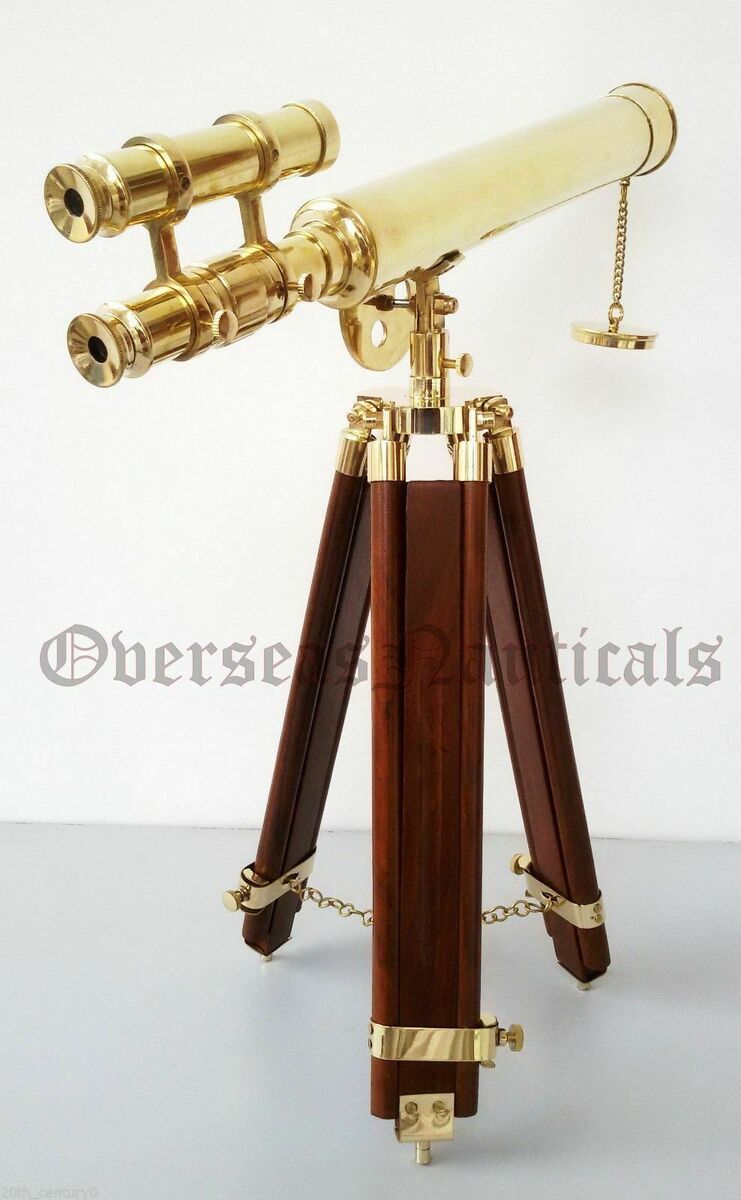The image displays a beautifully crafted vintage telescope, elegantly designed with a blend of gold and wooden elements. The telescope, which is predominantly brass, features an intricately detailed structure, highlighted by a hanging brass lens cap on a chain. The long brass eyepiece and brass spotting scope emphasize its ornate design. Mounted on a dark wood tripod stand adorned with gold accents, the legs of the tripod are connected by a gold chain, ensuring stability. Despite the clear quality of the image, a watermark centrally located is partially obscured by the telescope, making it difficult to read. The scene is set against a minimalist background with a gray floor and a white wall, suggesting the telescope might be a showpiece within a showroom.